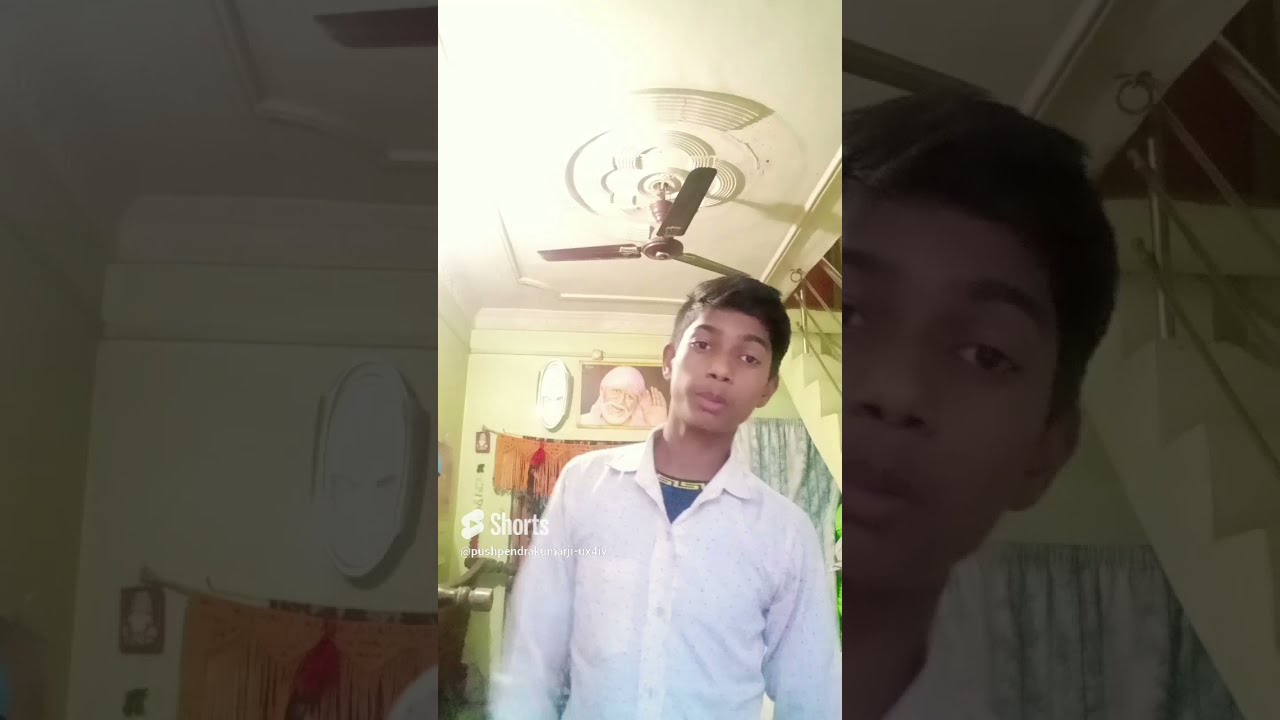The image is a vertical cell phone picture with a central focus on a young boy standing in an indoor room. He's wearing a white button-up shirt over a blue t-shirt, and has a neutral expression with his head slightly tilted to the right. His hair, short around the sides and longer on top, is black.

In the background, there is a light green wall with a painting of an old man waving, set near the ceiling. Below the painting are some orange and light green curtains. Above the boy is a white ceiling with a brown ceiling fan. A string is visible hanging against the wall, from the left and going behind the boy's shoulder, with an orange cloth hanging from it.

The image also features two columns on the left and right sides, each showing a zoomed-in, faded portion of the central image. The left column focuses on the wall and background details, while the right column is a close-up of the boy's face. Additionally, there is white text that reads "shorts" near the boy’s left arm, with more text underneath that is too small to read clearly.